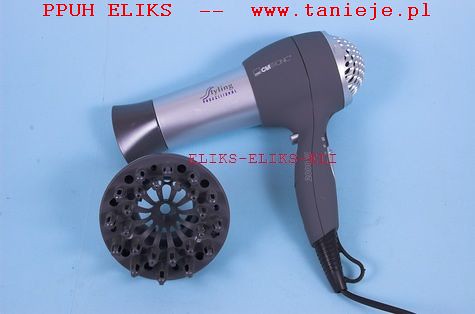This product photo showcases a hairdryer against a solid light blue background, which is about 30 to 50 percent wider than it is tall. The hairdryer is centrally placed and oriented at an approximate 8 o'clock position, with the power cord extending out towards the lower right corner of the image. The hairdryer features a matte black handle and main body, with a silver rear vent and barrel. The tip of the barrel, where the hot air is emitted, is black. A diffuser, which is a black circular object with holes, is positioned beside the hairdryer but not attached to it. There is a faint shadow underneath both the hairdryer and the diffuser. At the top of the image, in red text, it reads "P-P-U-H-E-L-I-K-S -- www.T-A-N-I-E-J-E.P-L," with additional text partially visible but blurred in the center of the photo.